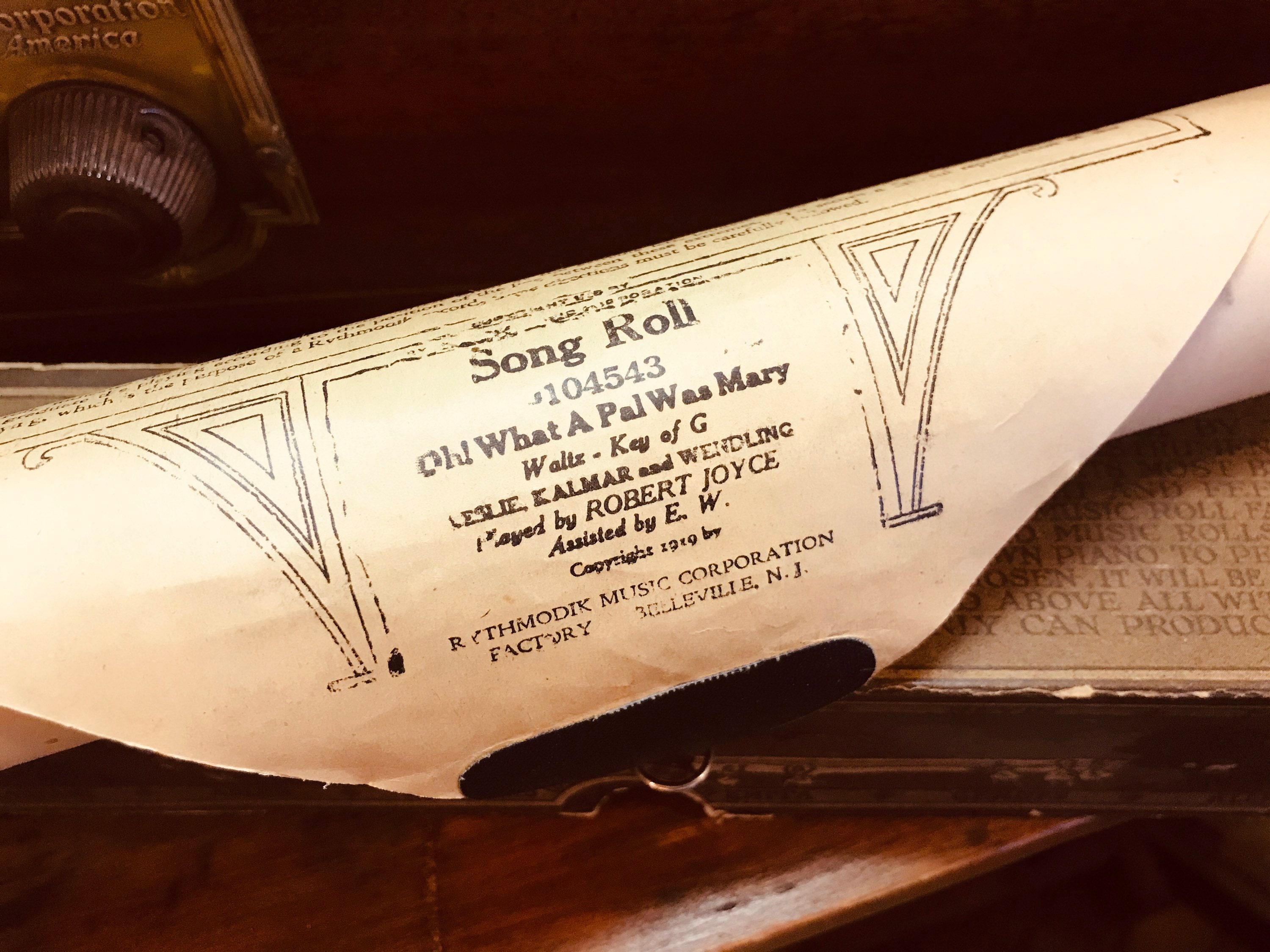The image depicts a partially unrolled white scroll of sheet music positioned in the middle of a vintage wooden desk, which has a dark reddish mahogany hue. The sheet music, printed with black text, prominently features the title "Song Roll 104543," followed by "Oh, What a Pal Was Mary, Waltz in Key of G." The credits attribute the piece to Robert T. Joyce, assisted by E.W., and note a copyright from 1929 by the Roth Modic Music Corporation Factory, Belleville, New Jersey. In the background, there's a glimpse of a possibly vintage appliance, such as a turntable or radio, indicated by a visible knob adjacent to the wooden surface. The overall setting suggests a recording studio or a historical music setup with a mix of pale white, black, rusty brown, and mahogany tones.